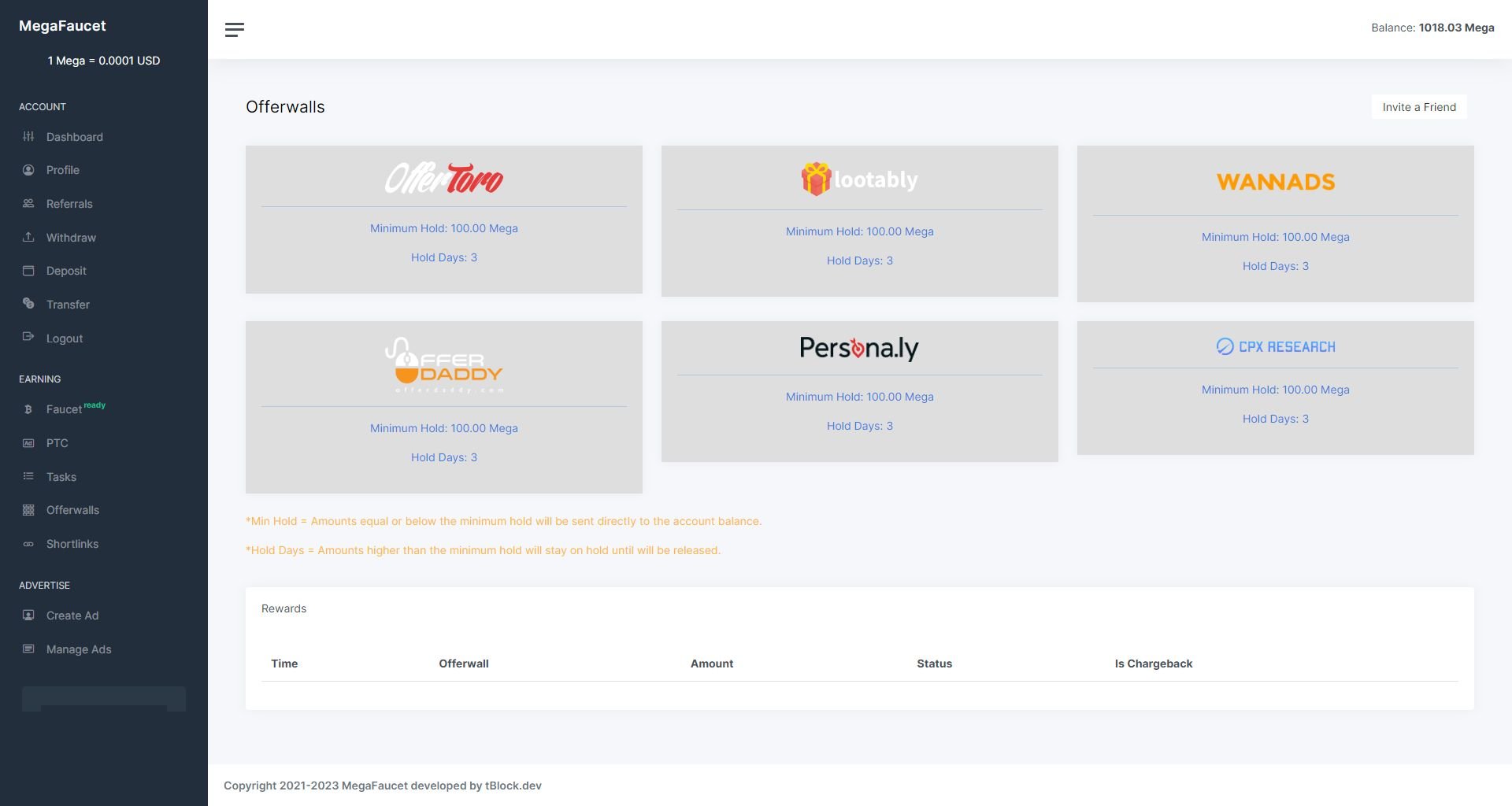The image depicts a detailed user interface of the Mega Faucet website. On the far left, there is a dark grey-blue navigation bar with text written in either white or grey. At the top of the bar, "Mega Faucet" is prominently displayed in white, followed by a note underneath stating "1 Mega equals 0.0001 USD."

Below the title, the navigation menu is segmented with the word "Account" in white, followed by various options in grey: Dashboard, Profile, Referrals, Withdrawal, Deposit, Transfer, and Logout. Each item has a corresponding icon to its left.

Further down, there are sections labeled "Earning," "Advertise," and more options below each, with text color-coded in white and grey. Notably, under "Earning," the items include: Faucet (with "Ready" in green next to it), PTC, Tasks, Other, Offer Walls, and Short Links, all with corresponding icons. Similarly, under "Advertise," the options listed are: Create Ad and Manage Ad, again each accompanied by icons.

Adjacent to the navigation bar is a white bar featuring three grey horizontal lines on the left and the text "Balance: 1,018.03 Mega" to the right. Below this, a section displays various offer walls, inviting users to engage with: Offer Toro, Lootably, Wanna Ad, Offer Daddy, Personality, and CPX Research. Each offer wall is illustrated in separate grey boxes with logos and supplementary information:
- Minimum Hold: 100.00 Mega
- Hold Days: 3

An orange-text note outside the grey boxes clarifies: "Minimum Hold = Amounts equal or below the Minimum Hold will be sent directly to Account Balance. Hold Days = Amounts higher than the Minimum Hold will stay on hold until released."

Towards the bottom, another white bar titled "Rewards" displays columns labeled: Time, Offerable Amounts, Status, and Is Charged Back, organized left to right.

Finally, at the very bottom of the page, in grey writing, the copyright notice reads: "Copyright 2021-2023 Mega Faucet Developed by T-Block Dev."